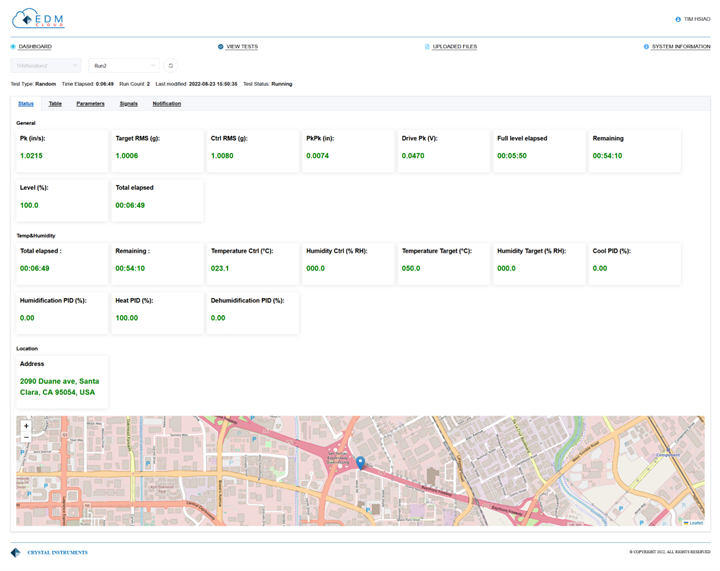The image depicts the desktop version of a website named "EDM something," which is notably not optimized for mobile viewing. The layout features a cluttered and visually unclear interface with particularly small text that makes interpretation challenging. The page seems to be displaying various data metrics, possibly related to a weather station located at 2090 Duane Avenue, Santa Clara, California, 95054 USA.

The upper section of the webpage lists a range of statistics including multiple timers, levels, and the total elapsed level, though their purpose is not immediately clear due to the small and difficult-to-read font. Additionally, there are various measurements displayed such as temperature, humidity, temperature target, humidity target, and cool PID percent, as well as information pertaining to humidification.

A GPS map is shown at the bottom of the site, marked by a pin at the provided address. Notably, the map carries a strange pink hue, which might indicate traffic conditions or some kind of environmental overlay. The ambiguous nature of the timers and other statistical data implies that the website's primary function may involve monitoring and presenting localized climate information, though the exact details remain ambiguous due to the website's poor design and illegible text.